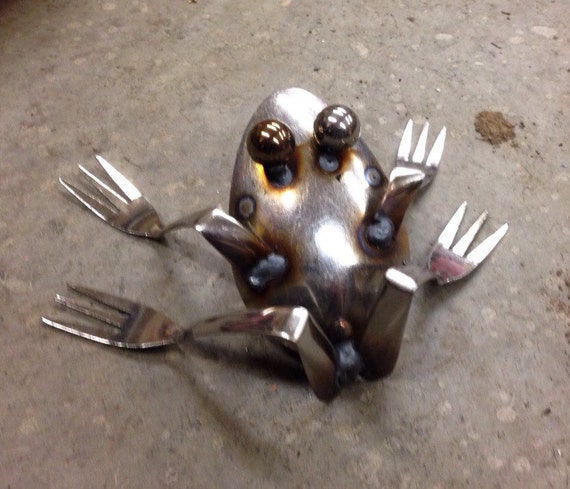The crafted object is a metal frog-like creature that appears to be handmade. The body of the frog is fashioned from the end of a polished silver spoon, while the limbs are formed from forks bent at angles slightly more than 90 degrees, approximately 100 degrees. Each fork, consisting of three prongs, serves as the frog's legs and arms, firmly welded to the spoon's mid-back area to mimic a frog's natural stance. The frog features spherical metal balls for eyes, giving it a lifelike appearance. The metallic frog is positioned on a gray, cement surface that is splotched with dirt and small patches, including a tiny piece of wood near its front limb on the right side. The frog's back faces the observer, with its attention directed forward, away from the viewer. The entire frog has a polished silver finish, adding to its shiny, artistic look.